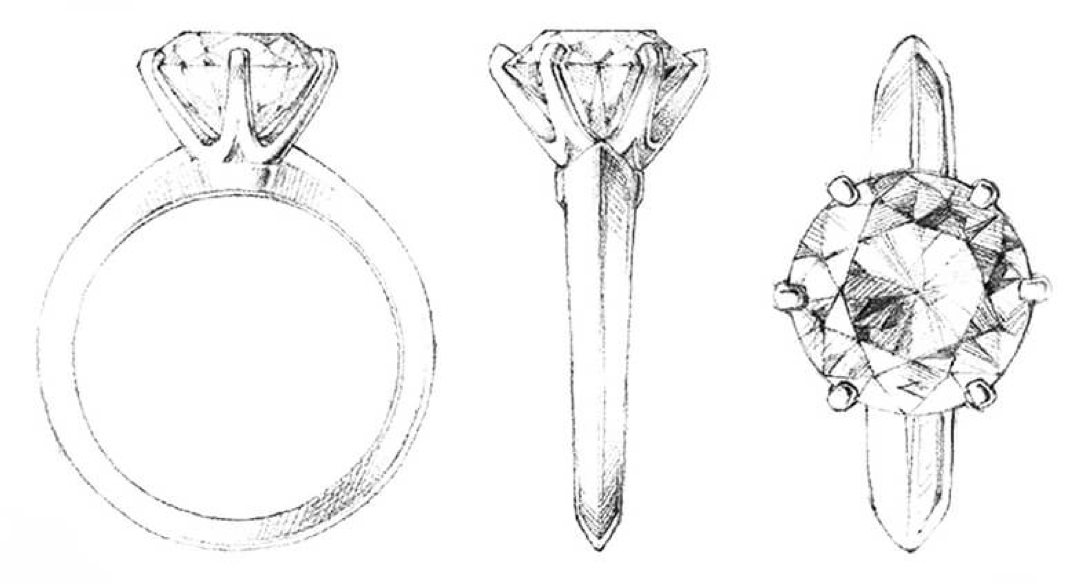The image is a detailed black and white sketch featuring three views of the same engagement ring on a white background, without a border or any text. On the left side, there's a faded depiction of the ring in profile, displaying the circular band with a diamond set on top. In the center, a more detailed side view highlights additional brackets or settings that secure the diamond, giving it a nail-like appearance. The right side presents a top-down view of the diamond, revealing six brackets holding the gemstone in place. The sketches collectively showcase different perspectives and intricate details of the ring's design, emphasizing the diamond and its secure setting.